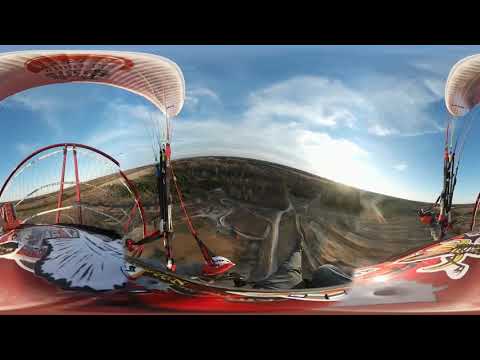The image is a small, horizontally aligned rectangular photo, framed by thick black borders at the top and bottom. The background is a blue sky adorned with wispy white clouds, with sunlight breaking through. Across the midsection, there's a curve of brown land leading to a green area, featuring trees and scattered roadways. Two distorted, narrow parasails or parachutes appear, one on the upper left and the other on the upper right, both linked to strings. The left parasail is white with a faint red logo in the center, while the right one appears primarily white. Below these parasails, there's a red area with white and black markings, but the image's severe blurriness and distortion make it challenging to identify. The ground beneath the parasails showcases a green terrain with an expansive field and some visible roads. Overall, the photo captures a high-altitude view, emphasizing a dynamic aerial scene, albeit relatively out of focus.